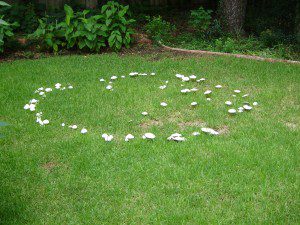The image captures a bright daytime scene in what appears to be a privately owned backyard. The foreground reveals a patchy yard covered in uneven green grass interspersed with small areas of dirt. Along the right edge of the scene, a border of some sort, possibly landscaping stone, delineates the yard from the background. Behind this border, there are various plants and a possibly single tree trunk standing amongst a bed of dirt or mulch. This backyard backdrop gives way to darker, more densely packed foliage, hinting at a line of trees or a forested area beyond.

In the middle of the yard, there is a notable formation: a circle of white mushrooms. These mushrooms range in size from very small to somewhat larger, with many forming an imperfect ring and others scattered towards the center of this circle. The mushrooms are predominantly white-capped and resemble varieties such as button mushrooms. Estimated to be between 30 and 40 in number, these mushrooms intriguingly create a distinct circular pattern amidst the patchy grass and sporadic dirt patches.